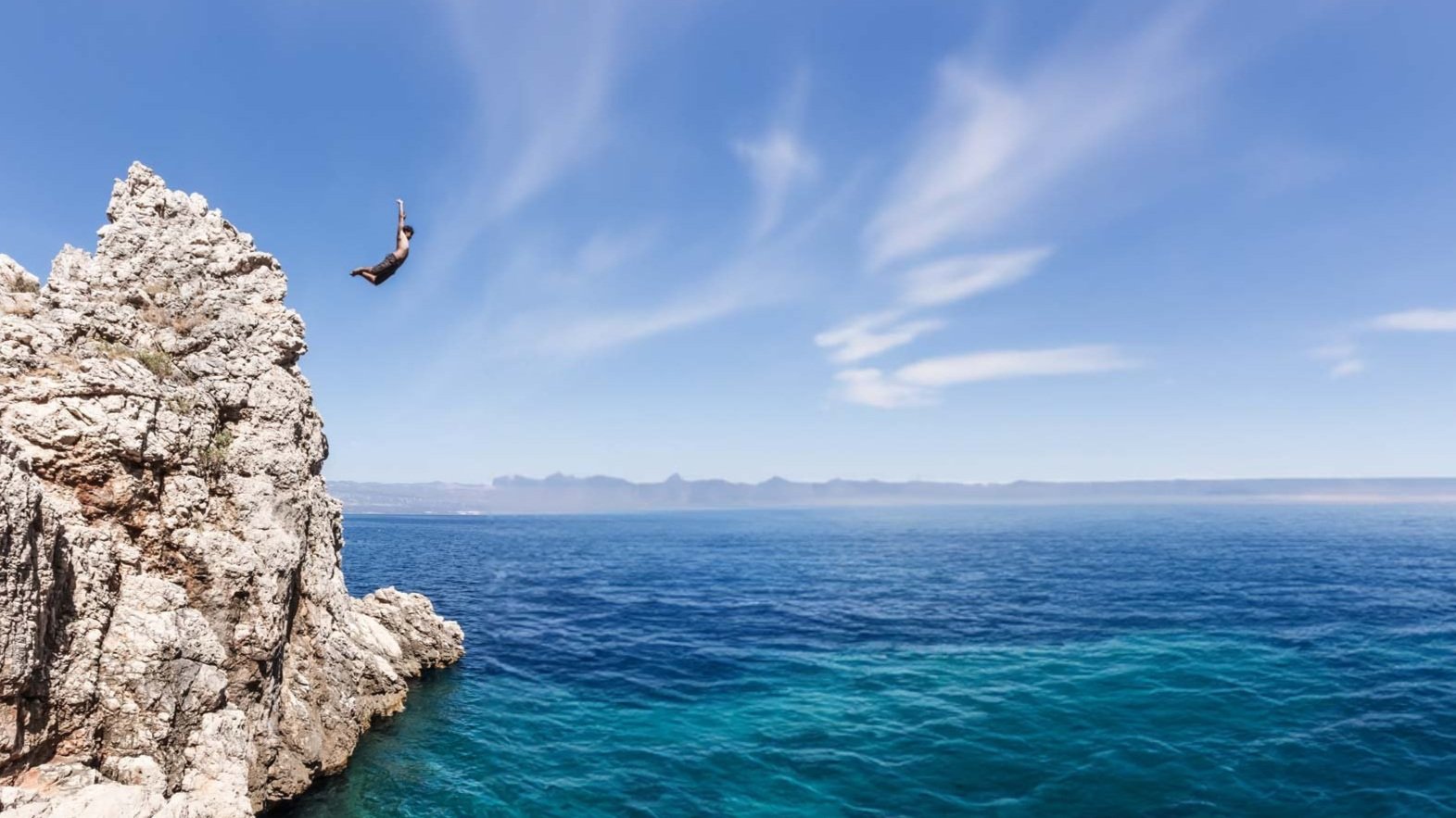A breathtaking wide-angle lens photograph captures a stunning coastal scene on a sunny day. The ocean waters below are a mesmerizing gradient of turquoise near the shore, transitioning to cobalt blue at the horizon. On the left side of the image, an imposing, irregularly shaped, bumpy rock cliff stands prominently. A daring man, wearing black swimming trunks, is captured mid-flight as he leaps off the tall cliff with his arms thrust above his head and his feet trailing behind him, poised more for a dramatic jump—perhaps a belly flop—rather than a precise dive. In the background, a line of low cliffs or possible mountains traces the horizon, while wispy white clouds streak across a perfectly blue sky. The scene is both thrilling and serene, perfectly encapsulating the raw beauty and adventurous spirit of the ocean landscape.